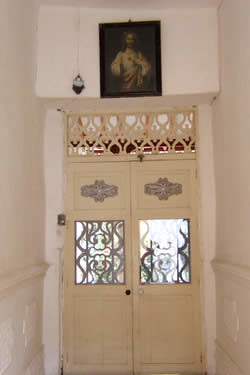This photograph captures an indoor scene of a distinctly high-ceilinged room, likely in a church, characterized by its off-white, plaster or concrete walls. The focal point of the image is a set of very old-looking double doors, exuding a sense of antiquity. The doors, painted in an off-white or cream hue, possess a rather unique composition. They are adorned at the top with intricate cross designs and feature central glass panels protected by ornate security bars. The lower sections of the doors are comprised of smooth, plain panels.

The left door is equipped with a black doorknob, while the right has a white one, suggesting a history of repairs or replacements. Above these doors, a small mesh opening allows for airflow, typical of arid climates. Crowning the doorway is a distinguished picture of Jesus Christ, adding a sacred aura to the scene. Additional details include white sconces affixed to each side of the entrance at the bottom, and the subtle presence of a baseboard running along the bottom edge of the scene. The overall height and scale of the room, coupled with these detailed features, enhance the sense of reverence and historical significance of the space.